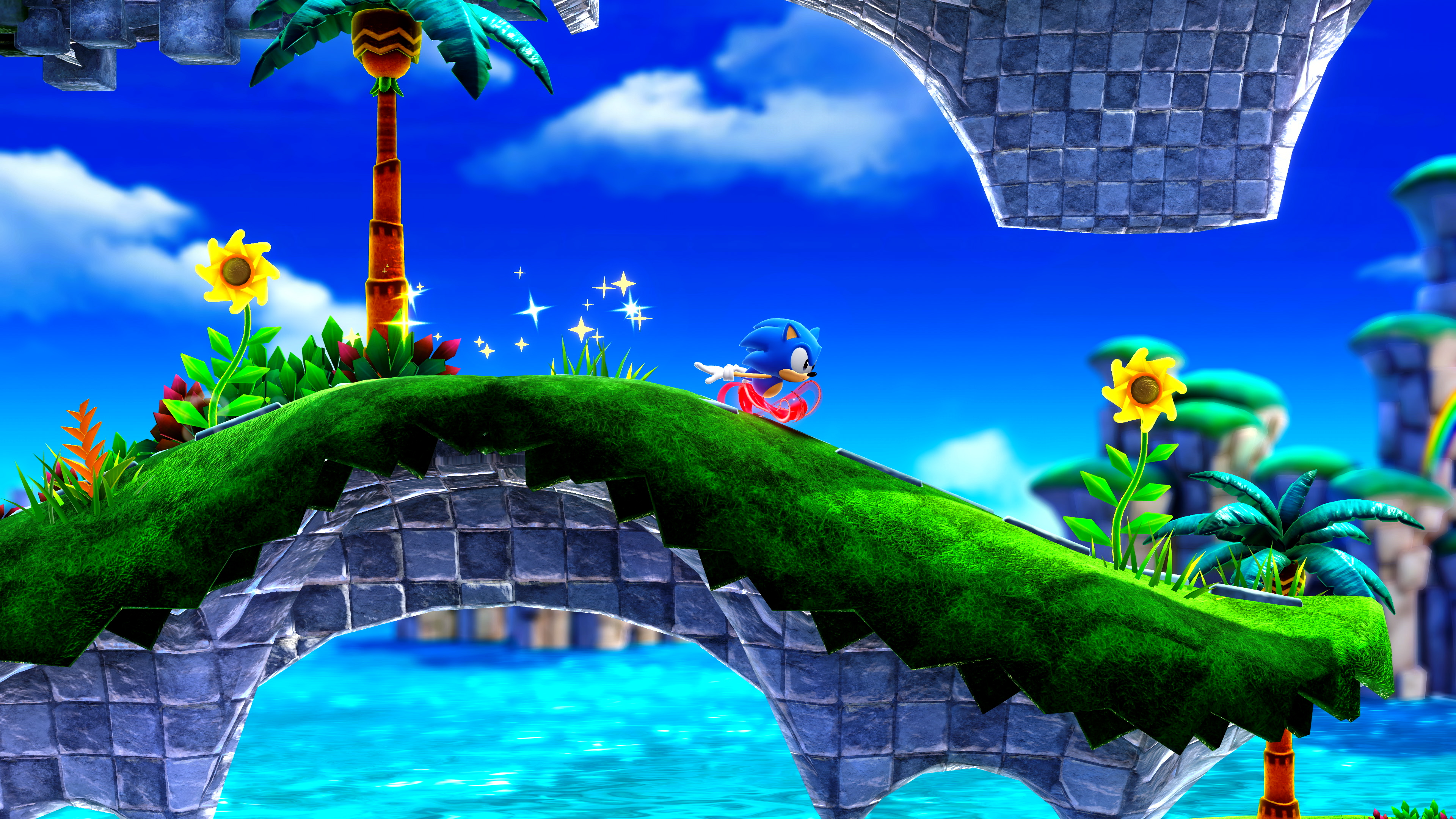The image depicts Sonic the Hedgehog, mid-run on a vibrant, computer-generated landscape typical of a video game setting. Sonic, characterized by his iconic blue color, red shoes, and white gloves, is speeding across a grassy, stone bridge set high above a body of water. His rapid movement blurs his legs into an indistinct flurry, leaving a trail of sparkly stardust behind him. The bridge, supported by rocks, features a mix of gray and dark gray checkerboard patterns and an arch cut beneath it. The lush green grass on the bridge is adorned with a yellow-orange sunflower in the front and another behind him, as well as a palm tree. The scene is set against a backdrop of bright blue sky dotted with a couple of wispy white clouds. In the distance, there's a landscape with small islands or grassy hilltops, and a faint rainbow arc gracing the bottom right corner, adding to the colorful, animated charm of the image.